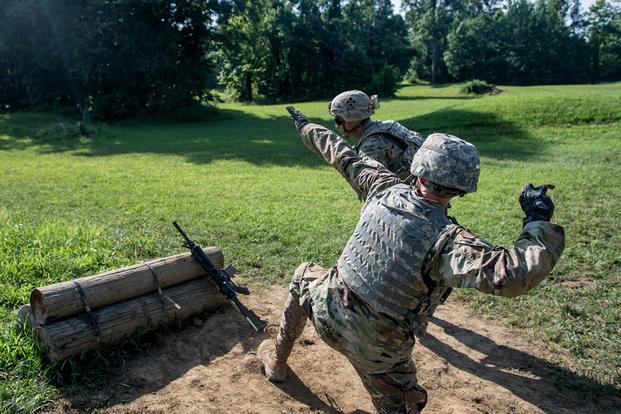In the foreground of this color photograph, two men dressed in military camouflage uniforms and bulletproof vests are captured in action. They are both wearing helmets and sturdy boots, suggesting they are engaged in a tactical exercise. The man closest to the camera has his back turned, one arm extended in front and the other drawn back as if he's about to throw a grenade. Parallel to the ground, his fellow soldier is crouched down to his right, leaning forward with his hands on his knees, intently gazing off to the left. A semi-automatic rifle is propped up against a stack of three wooden logs positioned in the bottom left corner of the frame. The scene is set outdoors during the daytime, in a grassy field bordered by dark, fully bloomed trees with patches of light blue sky visible through the foliage. The exact target or purpose of their action remains unclear, adding an element of suspense to the image.